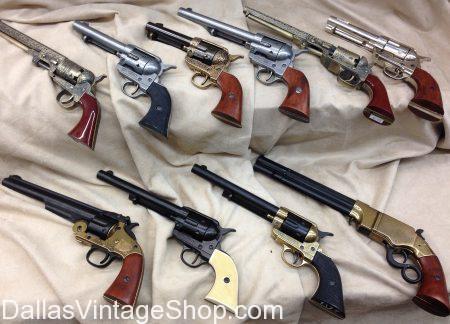This photograph showcases a collection of ten vintage, Western-style guns meticulously displayed on a slightly ruffled, off-white blanket. The arrangement includes six smaller guns on the top row and four larger ones on the bottom row. Each gun features intricate details, with some barrels adorned with decorative engravings and others featuring brass or gold-colored metals on their handles. The handles come in a variety of colors, including wood, ivory, and black. The entire collection is set against a tan-colored cloth, likely covering a table. At the bottom left corner of the image, the watermark "DallasVintageShop.com" is visible.